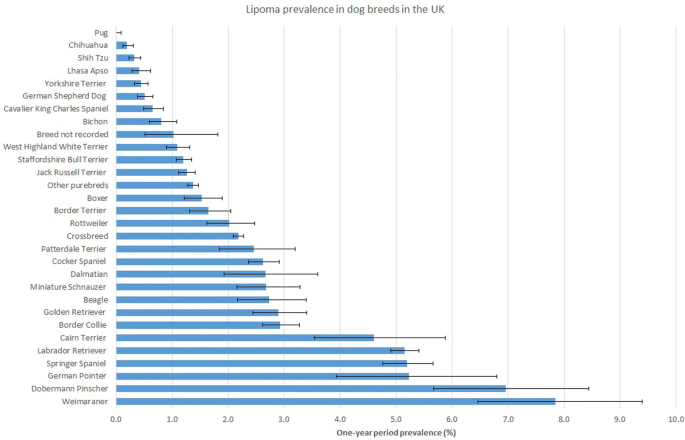This is a detailed graph titled "Lipoma Prevalence in Dog Breeds in the UK," illustrating the one-year period prevalence percentage of lipomas across various dog breeds. The horizontal axis ranges from 0% to 10%, while the vertical axis lists approximately 20 to 30 dog breeds in descending order of prevalence. At the top, breeds like Pug, Chihuahua, Shih Tzu, Lhasa Apso, and Yorkshire Terrier show the lowest prevalence, with Pugs having almost no cases. As you move down the list, breeds such as Boxer, Rottweiler, Crossbreed, and Doberman Pinscher exhibit increasing percentages, culminating with the Weimaraner at the bottom, showing the highest prevalence at around 7.8%. Each breed is visually represented by a blue bar denoting the prevalence percentage, providing a clear comparison of lipoma risk among different dog breeds in the UK.